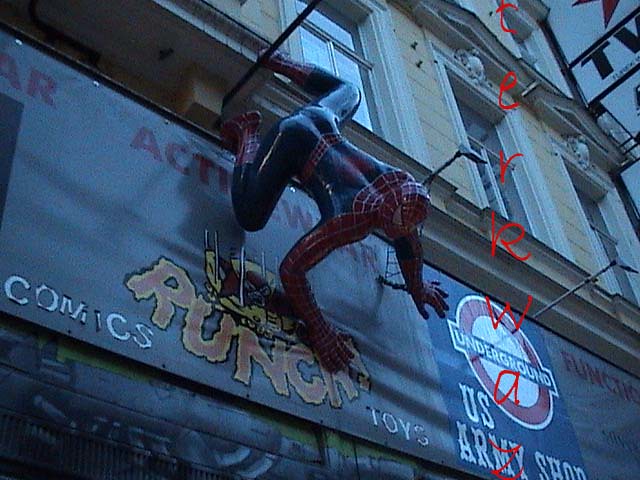In this detailed image, we observe a dynamic storefront scene prominently featuring a Spider-Man statue. The three-dimensional, solid sculpture of Spider-Man is affixed to a black bar, positioned as if he's crawling down towards the onlookers. His detailed suit is vividly painted: the head, shoulders, arms, upper back, and legs are adorned in striking red with intricate white web patterns, and large, triangular eyes. The rest of his costume, including the pants and chest, is a reflective blue, emphasizing the light shining off it. The statue is set against a dark gray banner beneath him, with the word "RUNCHY" emblazoned in orange letters, highlighted with yellow and green outlines. The lower left of the banner reads "comics," with "toys" and "U.S. Army Shop" positioned towards the right. Notably, red lettering spells out "TERKWAZ" from top to bottom on the right side. Above Spider-Man, the building façade features yellow walls with white-framed windows, adding to the scene's vibrancy. The image conveys a clear sense of action and intrigue, inviting patrons into what appears to be a themed comic and toy store, augmented with additional signs like "Underground" and "Jumper Web," enhancing the themed atmosphere of the old building.